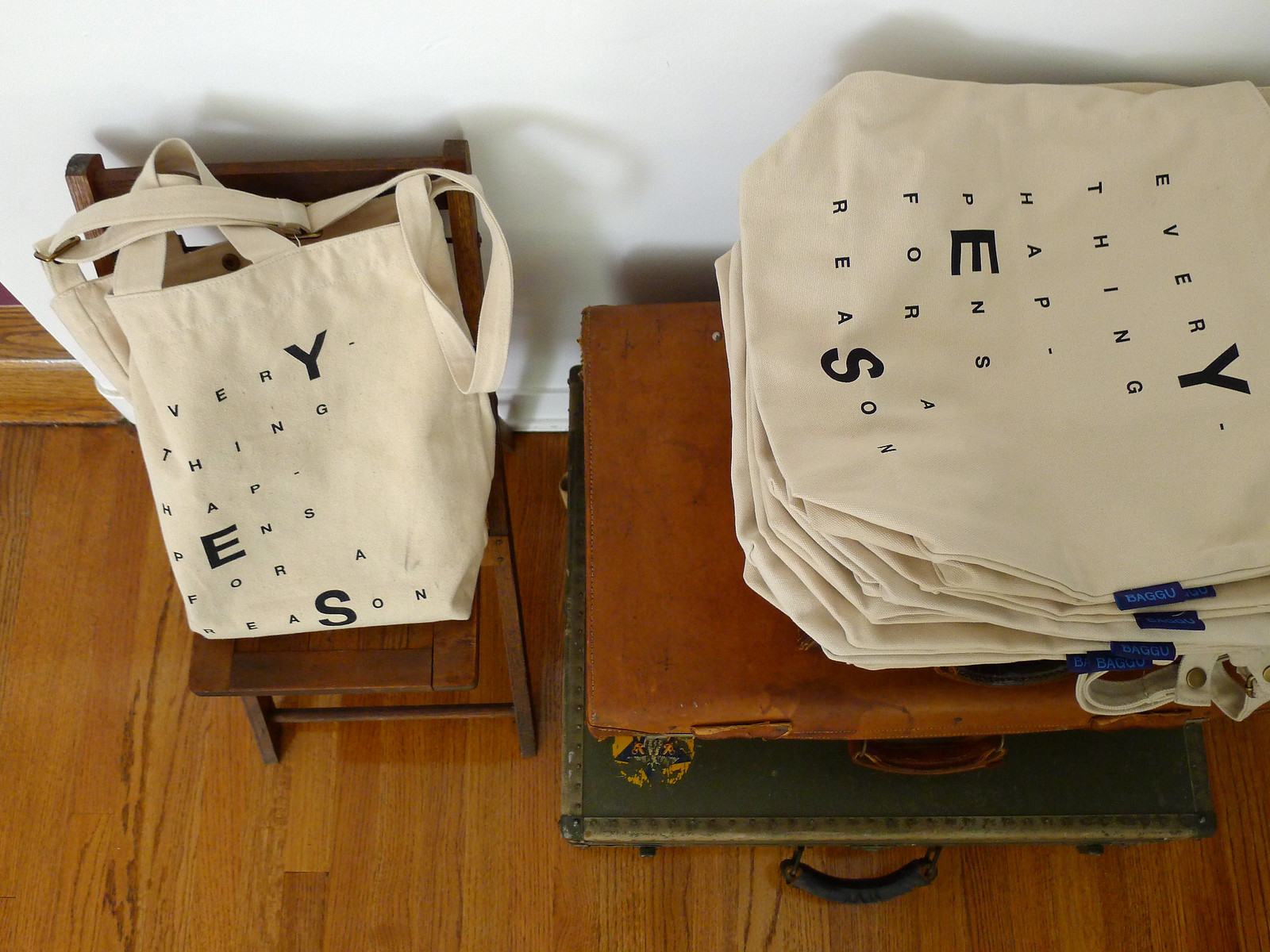The photograph depicts a quaint corner of a room with a wooden-paneled floor and a white wall. Leaning against the wall is a medium-dark wood folding chair with metal legs, which supports a beige fabric tote bag. The tote bag, with black text stating "Everything Happens for a Reason," highlights the letters 'Y,' 'E,' and 'S' in enlarged form. Nearby, there is a stack of identical tote bags, all sharing the same off-white, cream color. Below the chair, two stacked briefcases serve as makeshift shelves: one is a battered light to medium brown briefcase, and the other is a greenish suitcase with a handle, appearing hunter green in hue. The scene is well-lit, emphasizing the textures of the wooden floor, the fabric of the bags, and the worn surfaces of the briefcases.